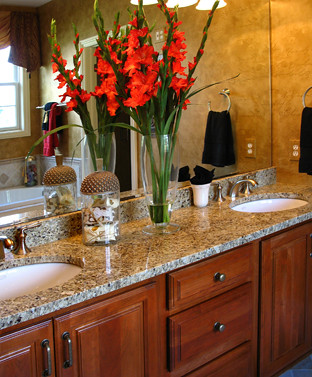The image displays a luxurious bathroom countertop fashioned from sleek, black and gray marble. The countertop houses two elegant white sinks paired with matte silver-gold faucets. Above the sinks, a large mirror is mounted on the wall, reflecting part of a bathtub and an array of additional towels hanging by it. 

On the left of the countertop, a vase brimming with red flowers stands tall, with blossoms tracing their way up the stems. Beside one of the sinks, there’s a cup containing a neatly rolled towel, adjacent to a decorative jar with a lid resembling a cactus, its contents indistinguishable.

A black hand towel hangs from the wall, conveniently placed near sink level. Beneath the counter, the wooden cabinetry adds a warm contrast, featuring knobs that gleam in the same silver-gold tone as the faucets. The bathroom's walls are painted in a coordinating gray-black hue, seamlessly blending with the marble countertop. Additionally, illuminated cabinets add a touch of brightness to the sophisticated ambiance, with visible outlets placed near the towels hanging on the wall.